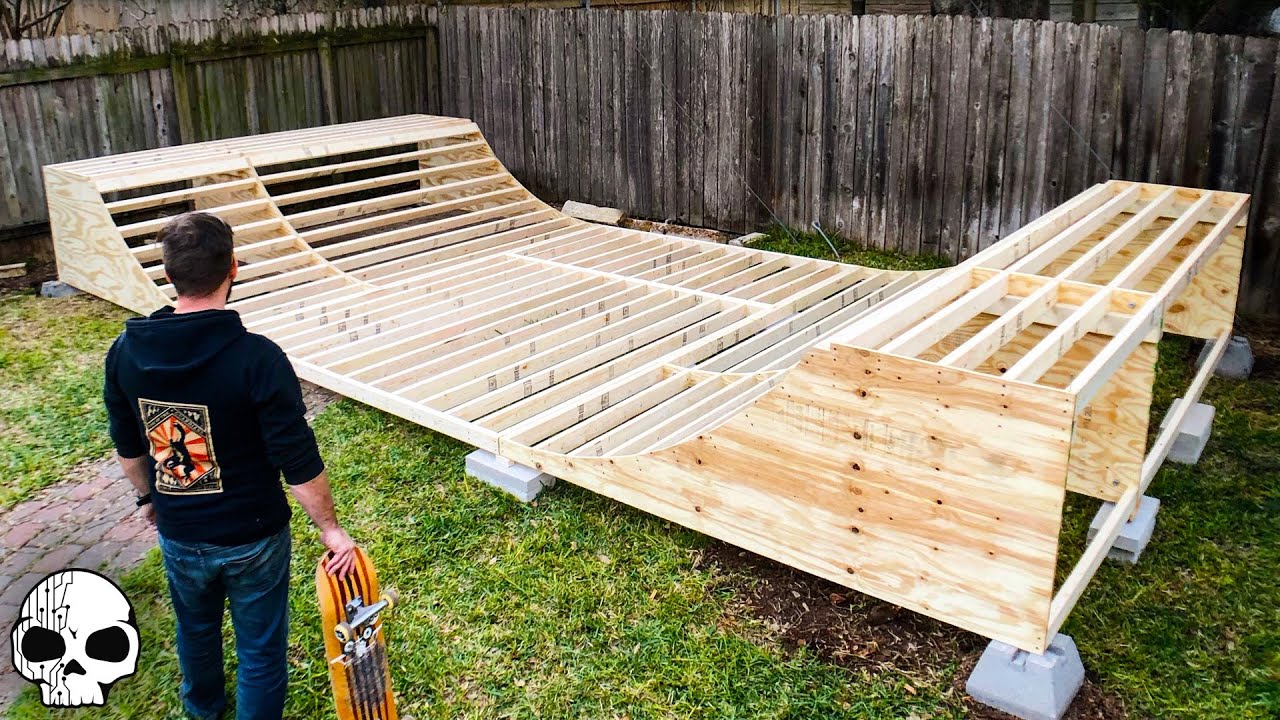This color photograph showcases a skater standing in a backyard, in front of an under-construction skateboard half-pipe. The half-pipe is made of unfinished light brown wood, revealing all the planks and supports without the final surface. This half-built ramp curves in the middle and rests on several concrete blocks. A dark grayish-brown wooden fence serves as a backdrop, juxtaposed with patches of green grass and a brick path seen in the bottom left corner, which also features a white stylized skull logo with numerous lines on the left side.

The skater, with short dark hair, is wearing blue shorts or denim jeans paired with a black hoodie that has an unspecified graphic or design on the back. He is facing the ramp while holding an orange skateboard in his right hand, which also features red and black elements. A wristwatch adorns his left wrist, adding to the casual yet focused skater persona presented in this detailed backyard scene.